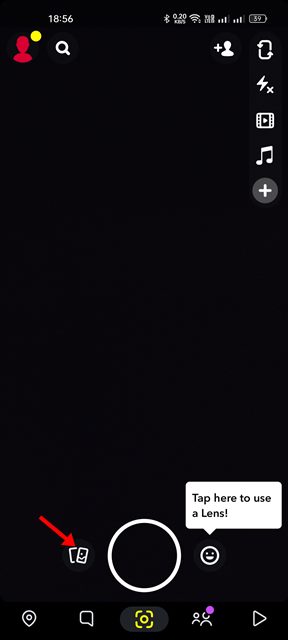The image displays a smartphone screen showcasing a primarily black interface with various icons and indicators. At the top, the time is shown as 18:56, accompanied by Wi-Fi and battery status icons. Dominating the upper section of the screen is a red outline of a human figure with a yellow symbol, suggesting some form of tracking or notification feature. Below this, search icon and an add button are visible, alongside multimedia icons for music, video, flash, and camera reversal, indicating the presence of both front and rear camera options.

Towards the bottom of the screen, an icon resembling two screens hints at a photo album or gallery. This is highlighted by a red pointer. Adjacent to it, there is a large white circle and a smiling face icon, with text prompting the user to "tap here to use a lens." The footer contains several icons: a location pin, a chat bubble, a central yellow circle (likely indicating the main action button), an icon depicting two people with a purple dot, and a send arrow.

Overall, this detailed interface appears to be part of an application running on the smartphone, blending elements of communication, media, and location functionalities.